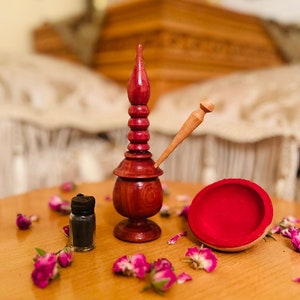The photograph showcases a highly ornate, polished wooden hookah designed in an Eastern style. The hookah is characterized by a round, ball-like base, resembling a tiered pagoda with four or five circular wooden rings ascending to a flame-shaped top where the smoking bowl is located. A tan-colored pin is inserted into the hookah, likely indicating the mouthpiece from where one inhales the smoke. The hookah sits prominently on a round, light wooden tabletop which is adorned with scattered purple and white flower petals. To the left, there is a clear glass vial with a black substance, capped with a black plastic lid. To the right, a salmon-colored dish, which might contain an incense powder, rests on the table. In the background, slightly out of focus, are curtains and wooden panels, further framing the central subject of the photograph. The overall image captures the intricate craftsmanship of the hookah and the serene setting it is placed in.